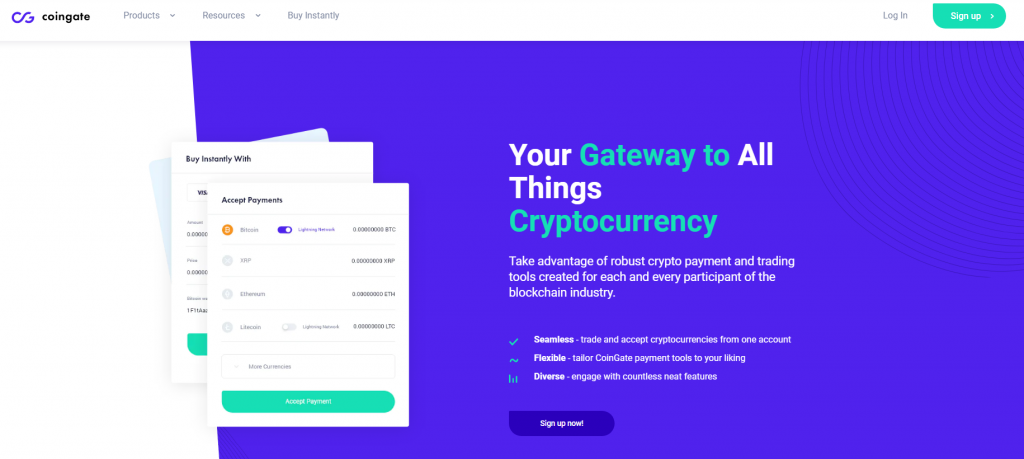The image features a clean blue background with a prominent blue box at the center. At the top, the header reads "CoinGate" in bold, followed by navigation options: "Products," "Resources," "Buy Instantly," and "Log In" / "Sign Up." 

Inside the blue box, the text "Your gateway to all things cryptocurrency" is displayed, with the words "gateway to" and "cryptocurrency" highlighted in green, and "your" and "all things" in white. Beneath this tagline, a descriptive line reads: "Take advantage of robust crypto payment and trading tools created for each and every participant of the blockchain industry."

Further down, three key features are listed with brief descriptions:
- "Seamless" - "Trade and accept cryptocurrencies from one account."
- "Flexible" - "Tailor CoinGate payment tools to your liking."
- "Diverse" - "Each with countless neat features."

Towards the bottom, a dark teal-colored box invites users to "Sign Up Now."

To the left side of the image, several white papers are visually represented, seemingly showcasing a few sample screens with the captions "Accept payments" and "Buy instantly with."